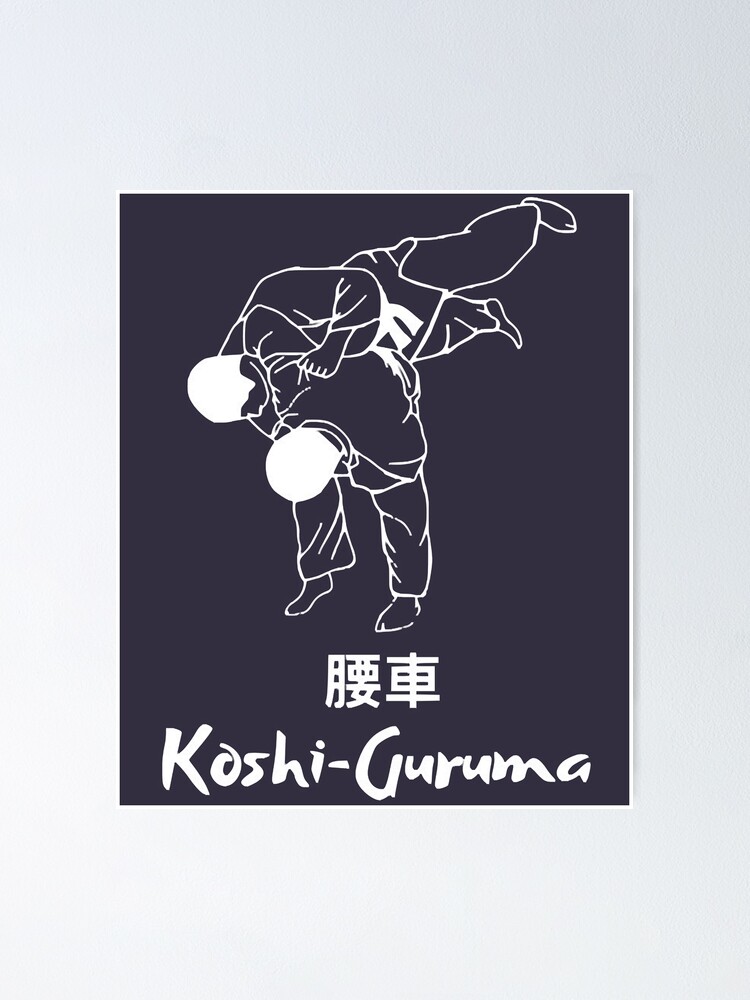In the center of this image, set against a minimalist black rectangle, two men are depicted in the midst of a dynamic karate move. One man, bent over, is flipping the other over his back, with the second man’s feet airborne and head pointing downwards, both clad in traditional karate outfits—cross-tied jackets and barefoot. The illustration is rendered in stark white silhouettes that contrast sharply against the black background. Framing this action scene is a thick white border, subtly shaded with dark gray hues on the right side. Above the men, there are Chinese characters, and directly below them are two blocks of white text. Additionally, in white, handwritten-like lettering beneath the text blocks, the title "Koshi Guruma" is prominently displayed, denoted as K-O-S-H-I-G-U-R-U-M-A, which translates to “waist wheel” — a nod to the depicted karate technique.